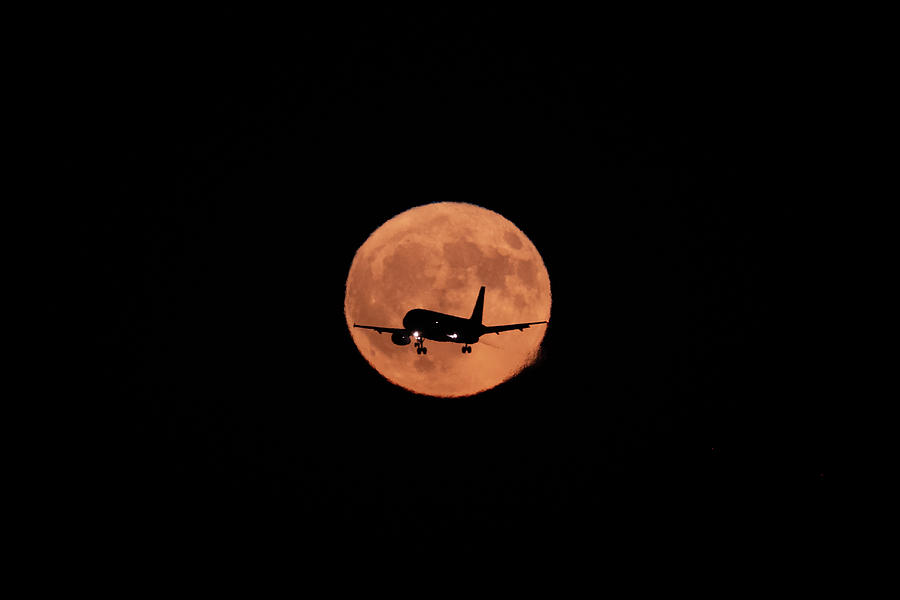This nighttime photograph captures a striking celestial event featuring a large, red blood moon dominating the sky amidst total darkness. At the very moment when a commercial airplane flies across the moon, the photographer captures the plane perfectly centered against the full moon. The moon appears in shades of light orange with light brown craters, contrasting against the pitch-black sky. The airplane, a black silhouette complete with its wings, tail, and still-engaged wheels, appears to be ascending, creating the illusion of flying dangerously close to—or even crashing into—the moon. The plane's bright white navigation lights punctuate the silhouette, adding compelling detail to this dramatic scene.